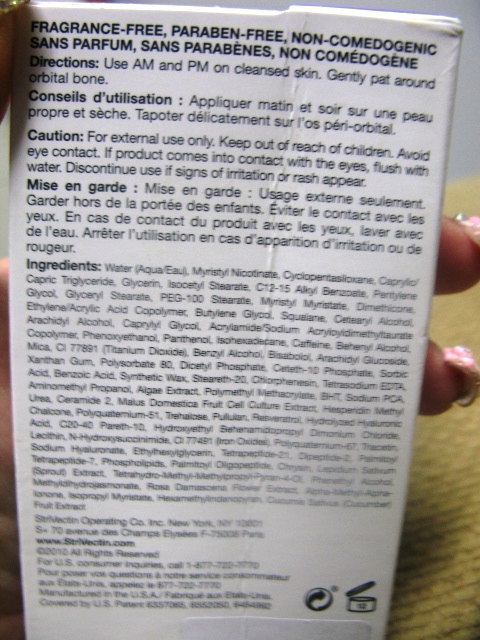In this image, a textured light brown table is set against a gray wall in the background. A woman's hands, with long fingernails painted a soft pink color, are prominently featured as she holds a product with a white label. The label, printed in black text, highlights the product's attributes: it is fragrance-free, paraben-free, and non-comedogenic. Additionally, the label provides usage instructions—apply both in the morning and at night on clean skin, gently patting around the orbital bone. Important cautionary notes are also included: the product is for external use only, should be kept out of reach of children, and contact with the eyes should be avoided. If eye contact occurs, the product should be flushed out with water, and use should be discontinued if irritation or rash appears.